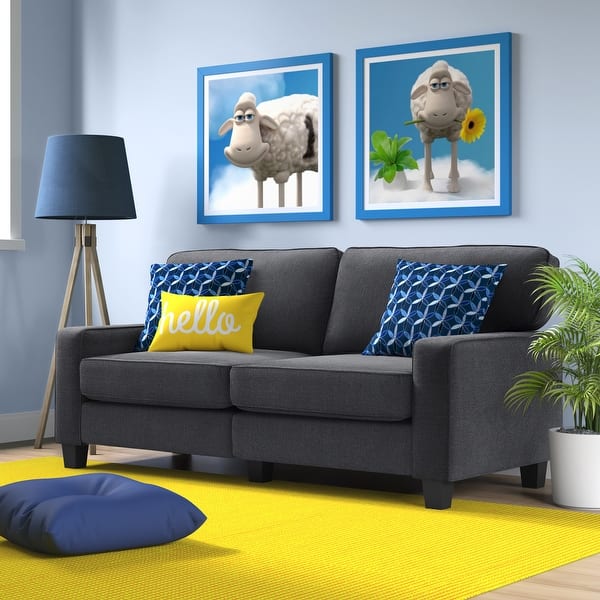The image depicts a cozy living room with a dark grey, two-seater sofa positioned centrally. The sofa is adorned with two blue pillows, one on each end, and a yellow pillow inscribed with "hello" in white cursive on the left side. Adjacent to the sofa on the left is a floor lamp with tan legs and a dark blue shade. To the right of the sofa stands a white pot holding a tall green plant. The backdrop features light grey walls with two square framed illustrations of sheep. One sheep looks directly at the viewer with a cheerful expression, while the other sheep, also facing forward, is holding a yellow flower in its mouth with a potted plant beside it. The floor is made of light hardwood, accentuated by a yellow rug.